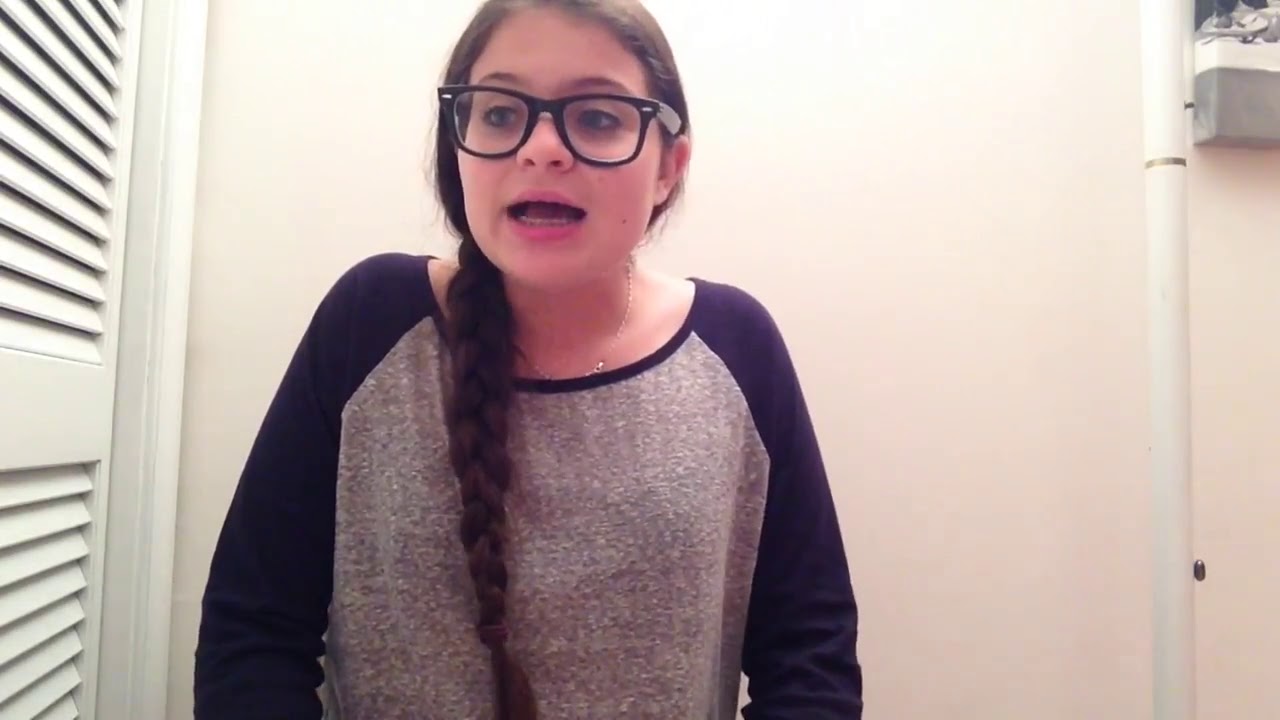This detailed image captures a young girl, possibly a teenager or tween, standing in a small, utility room or closet-like space. She has long, dark brown hair styled in a braid that hangs over her shoulder. She wears black-framed glasses with gray earpieces, and her mouth is open as if she's mid-speech. Her light skin contrasts with her gray, slightly baggy t-shirt featuring long blue raglan sleeves. Behind her, the off-white wall is bordered by a louvered door or window with blinds on the left. To her right, a tall white PVC pipe runs vertically up the wall, adjacent to a gray and white electrical box. The composition of the image highlights the snug and functional nature of the room.